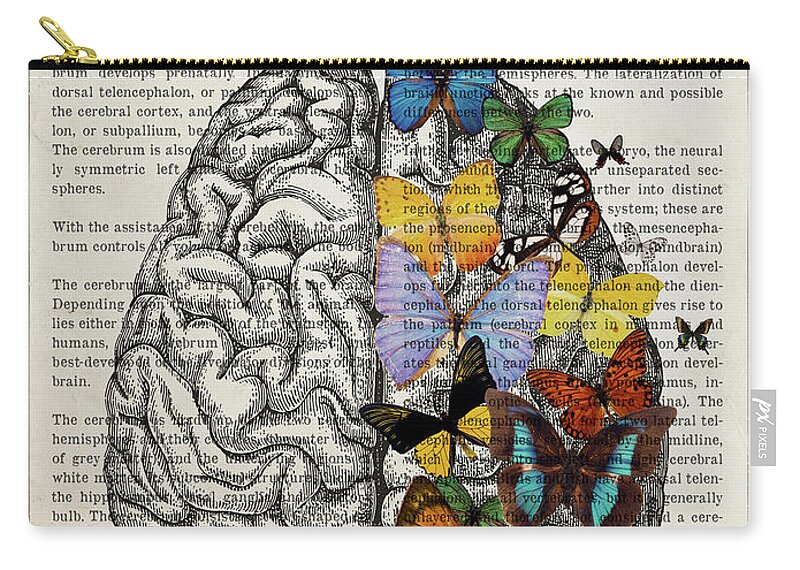The image depicts a pencil case with a digital collage design. The bag, which is primarily intended to store pencils, features a faux golden zipper running along the top. The background consists of a page from a book, where the text is partially obscured by a pen and ink drawing of a human brain. The brain's left side remains unembellished, showcasing its muscly, wavy texture, reminiscent of textbook illustrations. In striking contrast, the brain’s right side is adorned with an array of multicolored butterflies in shades of blue, green, yellow, purple, red, and brown. These butterflies vary in size, with some being small and others covering significant portions of the brain. This artistic design seems like a prototype image, possibly from PX Pixels, demonstrating how a customer's artwork would look when printed on the product. The combination of the intricate brain sketch and the colorful butterflies creates a visually appealing, layered composition.